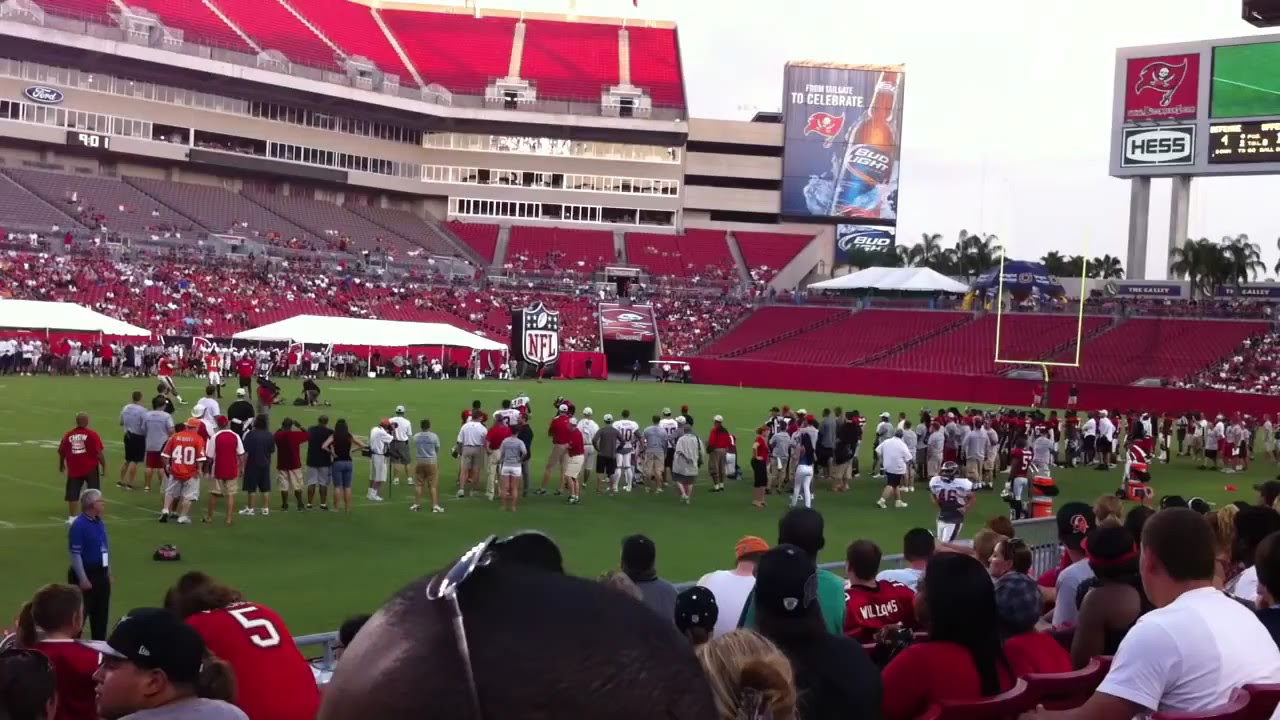The photograph showcases an outdoor event at the Tampa Bay Buccaneers' NFL football stadium, taken during daytime under a light sky. The view, captured from the stands, reveals a vivid green grass field where approximately 50 people have gathered, likely for a training camp practice. The stands, filled with a culturally diverse crowd dressed in red jerseys and shirts, are equipped with red chairs. Part of the stadium structure features many windows and is built on a gray concrete foundation, indicative of the suites. Palm trees can be seen in the distance, enhancing the Floridian ambiance. Several advertisements are visible, including a large Bud Light banner, a Ford logo, and an LED scoreboard displaying the Buccaneers' logo and an ad for HESS.